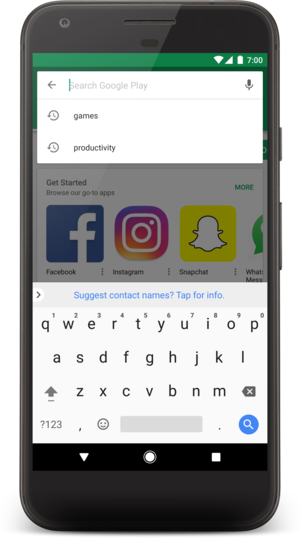The image depicts a cell phone displaying a screenshot of a Google Play search interface. The device shows it is exactly 7:00, with both the battery and Wi-Fi signals at full strength. The display features the Google Play search history, indicating previously searched categories like "games" and "productivity," though no current search is active. The bottom of the screen shows a keyboard for typing. The center of the screen prompts users to "Get Started" with options to browse or go to apps. Suggested apps include Facebook, Instagram, Snapchat, and WhatsApp Messenger, each accompanied by their respective icons. The phone itself appears to be an average model, with no visible branding that would indicate its make or manufacturer.